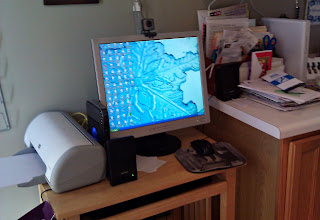In this image, we observe an individual working within an extremely limited space. The focal point is a small wooden table, roughly estimated at two feet in length and about 15 inches in width. This table features a pull-out tray intended for a keyboard beneath its surface. Atop the table sits a computer monitor, displaying a map with blue gradient colors as the desktop background. The desktop appears cluttered with numerous icons.

Additionally, the table supports a mousepad and speakers. To the left side of the table, a compact printer is positioned sideways, barely fitting within the tight area. Adjacent to the table, there is a cabinet with a Formica top. This cabinet is topped with stacks of correspondence and possibly some pictures, rendering the space even more congested.

The entire setup is nestled against a wall, where a picture frame hangs above, its details unclear. The overall arrangement evokes the imagery of a typical student's dorm room, characterized by its minimal and highly compact space.